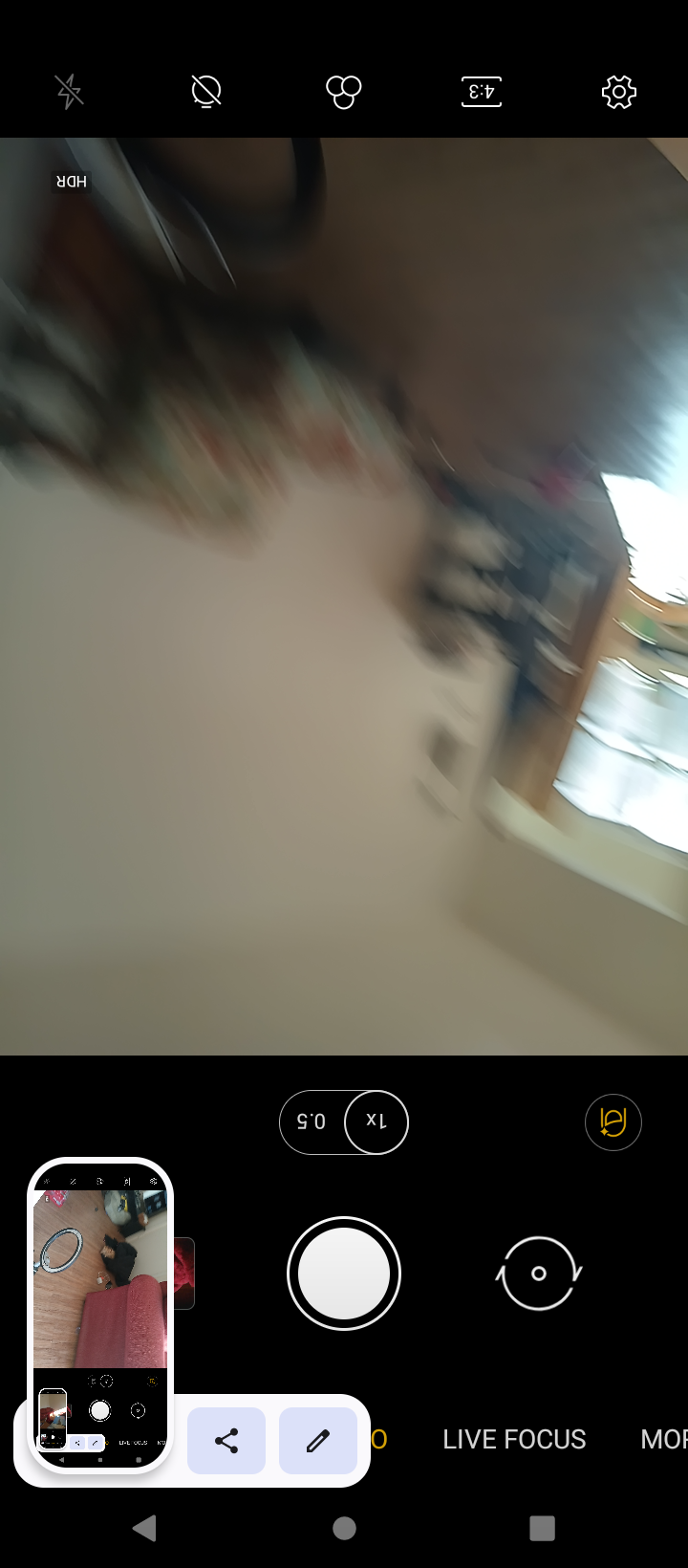This is an upside-down screenshot of a camera app interface, capturing a blurry image of what appears to be a room. The room has off-white walls, a window, and brown flooring. There is also a faint image of a black chair. The right side of the screen shows a blurred white object, possibly a cat, with black and brown items behind it illuminated by white lights. At the bottom of the screenshot, various phone symbols, such as the flash, settings, and HDR icons, appear inverted. The image also displays "Live Focus" in black text on a black background, with a white circle indicating 1x magnification and 0.5x in an expanded circle. A smaller inset picture, different from the main image, is located on the left side, showing something red. Along the bottom of the app interface are buttons for sharing, editing, and Live Focus, plus an additional text beginning with "MO" that is partially visible.